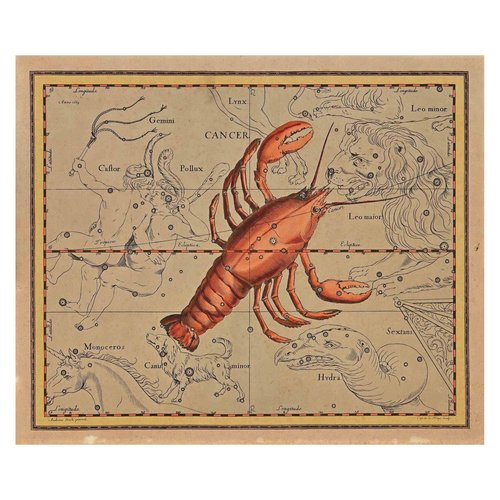This intricate, hand-drawn celestial map, set against a white background, features a vivid orangey-pink lobster at its center, angled at 45 degrees with its tail pointing to the lower left and its head to the upper right. The lobster, depicted with its characteristic claws and segmented body, is labeled as Cancer, representing the astrological sign. The map is bordered in beige with gold trim, while all text is rendered in brown, enhancing its antique appearance.

Surrounding the lobster, various constellations are meticulously illustrated. To the top right, Leo Major and Leo Minor are represented by a large lion's head and front paws, respectively. The left side of the lobster hosts Gemini, with Castor wielding a whip and Pollux holding a club. Directly above the lobster's left claw, the Lynx constellation shows a quadruped's hind legs.

Beneath the lobster’s tail, Canis Minor, a small dog, is drawn, and further left, the unicorn constellation Monoceros appears with its head, neck, horn, and upper back. Below the lobster's right claw, Hydra emerges as a snake-like creature with a bird-like beak. Far right, the map displays Sextans, a constellation represented by a geometric corner.

This detailed map, evocative of historical astrological and astronomical charts, likely spans over a century in age and provides a fascinating blend of mythological creatures and constellations.